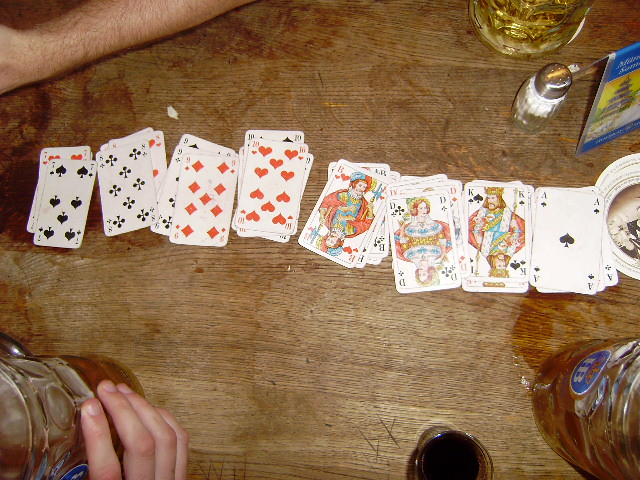In the image, a rustic, well-worn table serves as the backdrop for a casual scene. Sprawled across the wooden surface is a collection of playing cards meticulously organized into groups, with aces, kings, queens, jacks, tens, nines, fives, and sevens each piled separately. Every suit within these groups is represented, hinting at a card game that perhaps requires a selective assortment of the deck.

A hairy arm rests on the table, suggesting a relaxed posture, while another hand grips a glass, mid-sip, indicating someone enjoying a drink. Nearby, a salt and pepper shaker duo stands close to a water bottle and a small, dark jar that likely contains soy sauce. Directly in front of the glass-holding hand is a petite plate, adding to the lived-in feel of the scene.

The table itself is noticeably worn, its surface marked with the character of countless past gatherings and games. This assemblage of everyday objects conjures a vivid snapshot of a moment steeped in casual camaraderie and simple pleasures.